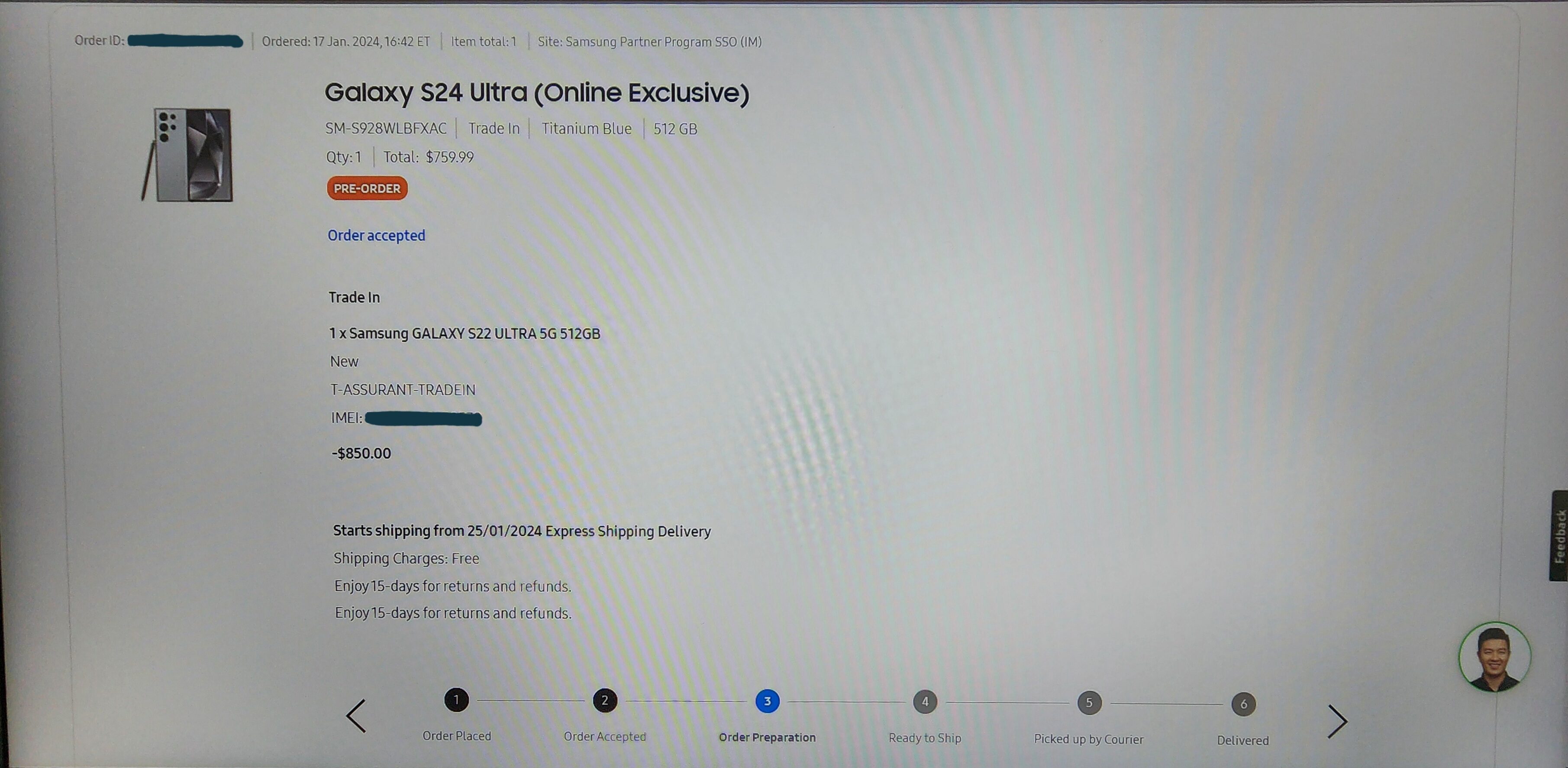Set against a solid white background, the image is a photo capturing a somewhat skewed screenshot of an online order summary. The displayed screen details a specific order with the following information: 

- Order ID
- Ordered on January 17, 2024, at 16:42 Eastern Time
- Item Total: 1
- Site: Samsung Partner Program SSO

Prominently featured in bold black text is "Galaxy S24 Ultra, Online Exclusive." Beneath that, in smaller gray text, is the product code, "SM-S928," along with "WLB-FXAC, Trade-In Titanium Blue," indicating the color and trade-in details, and "512 GBs, Quantity 1, Total $759.99," denoting the storage capacity and order cost.

An action button below in bright orange reads "Pre-Order." Adjacent to the button, in blue text, is the status update "Order Accepted."

To the left of this textual information, there is an image of the Galaxy S24 Ultra. Additionally, a trade-in value for a Samsung Galaxy S22 Ultra 5G, 512 GB, is noted, showing a deduction of $850 from the total.